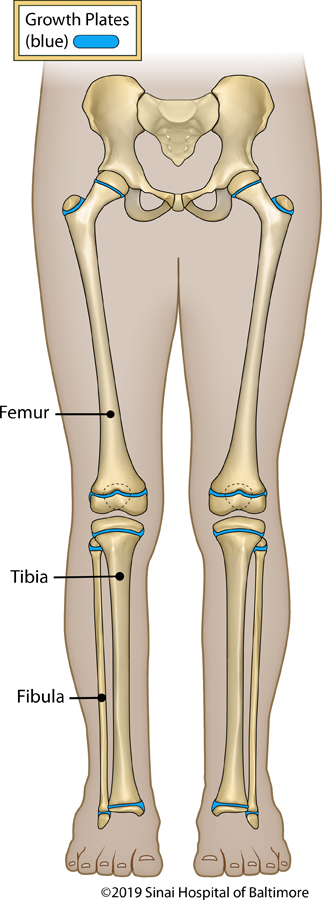This image is a detailed, portrait-oriented diagram of the lower half of a human body, viewed from the waist down to the feet, against a plain white background with no visible borders. The diagram highlights the bone structure in an off-white bone color, emphasizing the pelvis, femurs, tibias, and fibulas, each labeled accordingly. Notably, the bones of the feet are not included. At the upper left-hand corner, there is a small white rectangle with a gold outline, containing black text that reads "growth plates" with a blue oval adjacent to it, signifying that blue lines indicate growth plates within the diagram. These blue lines are visible at the key joints, including the hips, knees, and ankle areas. Additionally, a copyright notice at the bottom right corner in black print reads "© 2019 Sinai Hospital of Baltimore." This visual aid effectively illustrates bone growth plates and their locations within the lower limbs.